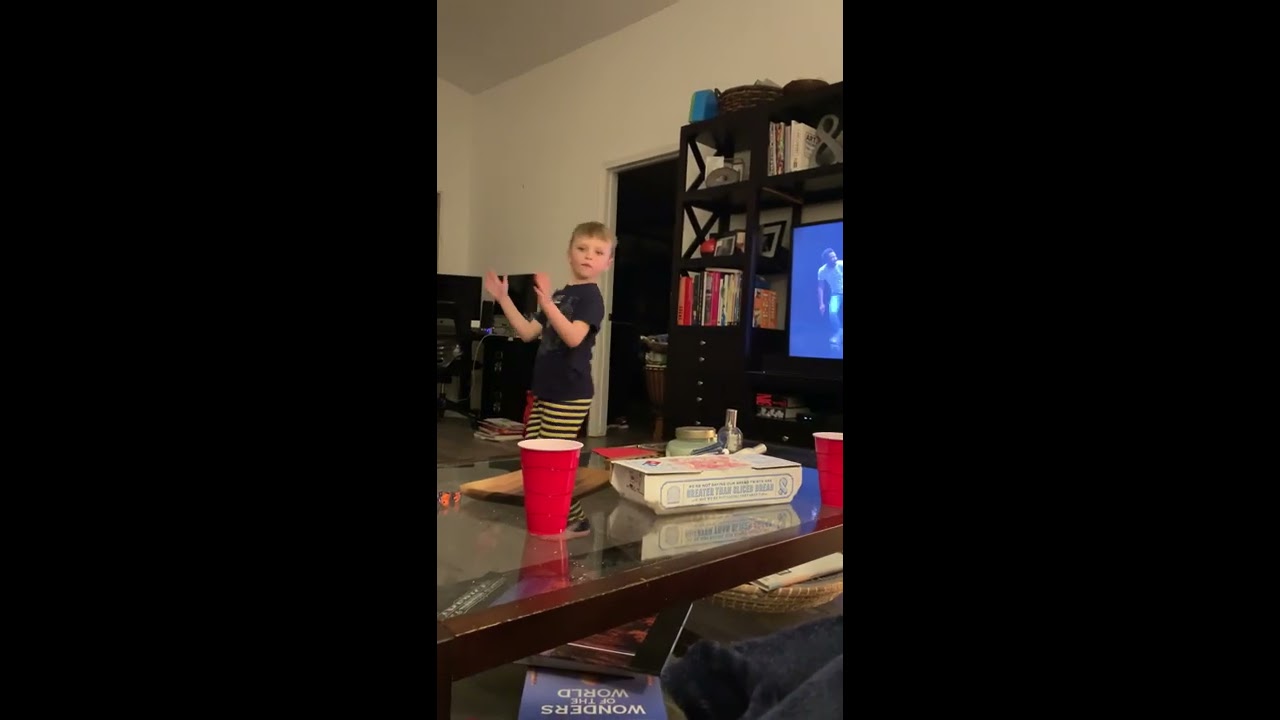In the living room, a boy with dirty blonde hair, dressed in a black t-shirt and yellow and black horizontal striped pants, stands with his body facing about 9 o'clock while looking neutrally at the camera. His hands are raised to chest level, elbows bent at 90 degrees. In the foreground, a glass coffee table with a brown trim holds a pizza delivery box, likely from Domino's, and red Solo cups. Below the table, a basket and several books are visible, including one titled "Wonders of the World." To the right of the boy, an entertainment stand houses a flat panel TV, which is on, along with numerous books and other items on the shelves. The room's off-white walls and gray ceiling provide a neutral backdrop. Additionally, there's a desk with a computer in one corner and an open doorway behind the boy, adding depth to the living space.